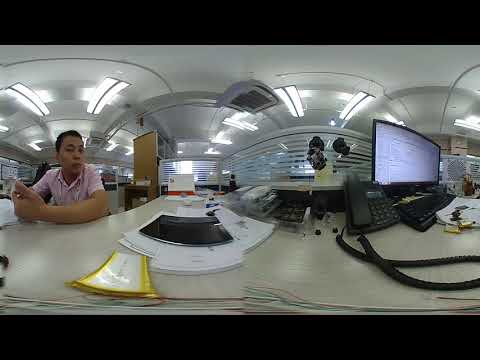This image captures an interior scene of a nondescript office space featuring a predominantly white and cream color palette. In the foreground, there is a cluttered white desk adorned with various items including a computer monitor, a keyboard, a telephone, and scattered paperwork. Situated towards the left-hand side of the image, an Asian gentleman with short brown hair and tan skin is seated at the desk, wearing a light pink collared shirt and resting his arms on the desktop. His facial expression suggests a lack of enthusiasm, adding to the overall impression of a low-energy, disorganized work environment. The background reveals more office elements like a curved gate area, windows, and a doorway, all illuminated by bright fluorescent lights from the ceiling. The scene exudes a sense of clutter and disarray, hinting at a less than productive atmosphere.